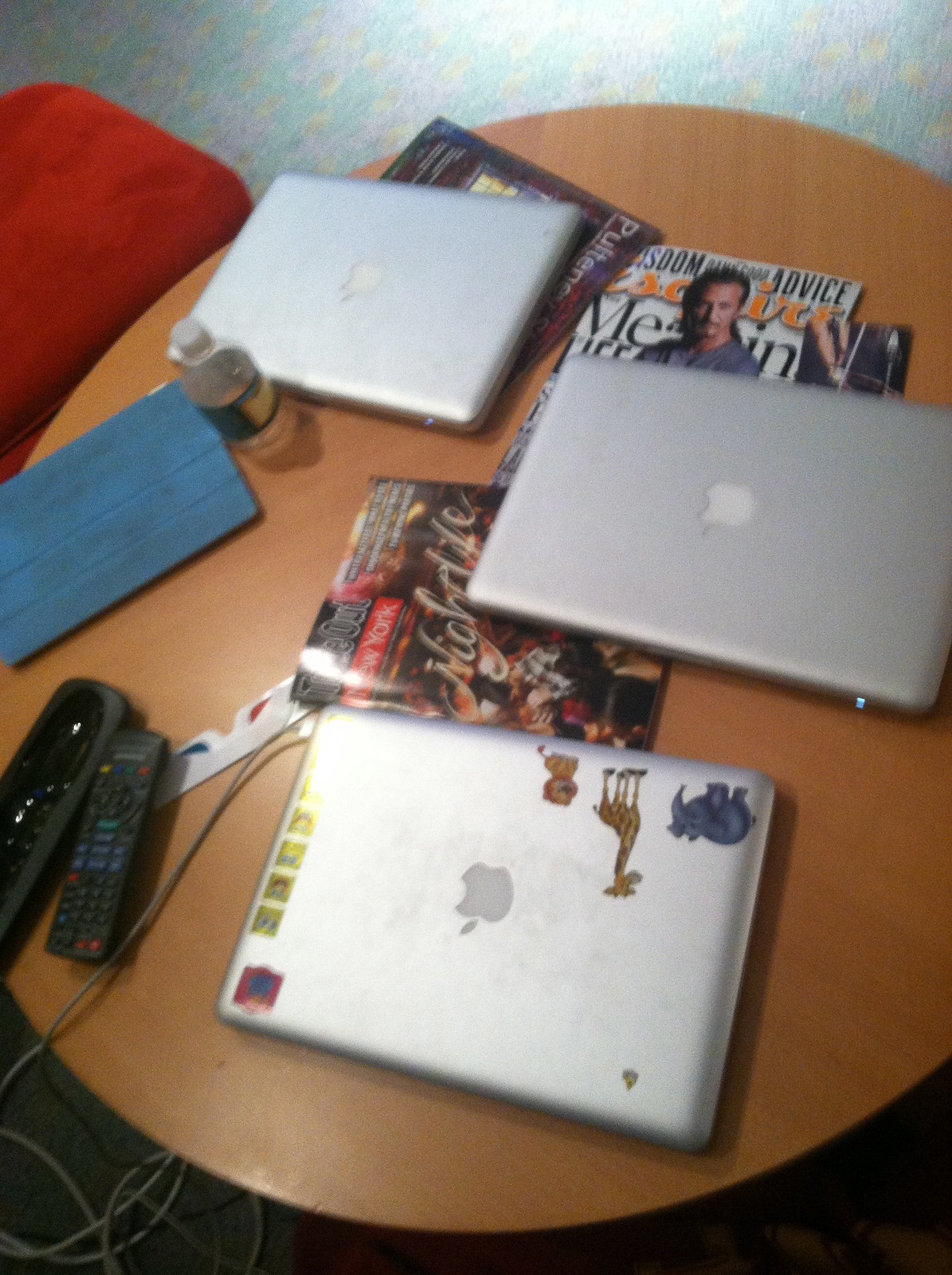The image depicts a slightly blurry scene centered around a large, circular wooden coffee table with a warm, orangey-brown hue, which appears to be situated in a dorm-like setting, atop a colorful carpet adorned with yellow dots. The table is cluttered with various items including three silver Apple MacBooks, one of which is decorated with stickers of a giraffe, an elephant, and a lion. The other two Macs are devoid of any stickers. Additionally, there are TV remotes with colorful buttons, a pair of 3D glasses, and an iPad encased in a fuzzy blue cover. Among the scattered items are several magazines: one identifiable as "Esquire," another detailed as "Time Out New York Nightlife," and a third partially visible with possibly the title "PULTENE" hinting at some vegetation imagery. A tangled charging cord is visible in the bottom left corner, connecting one of the laptops. Also on the table are a water bottle and a black item, likely a speaker or remote holder. In the upper right-hand corner of the image, a red piece of furniture, possibly a beanbag chair, is noticeable, adding to the overall collegiate vibe.